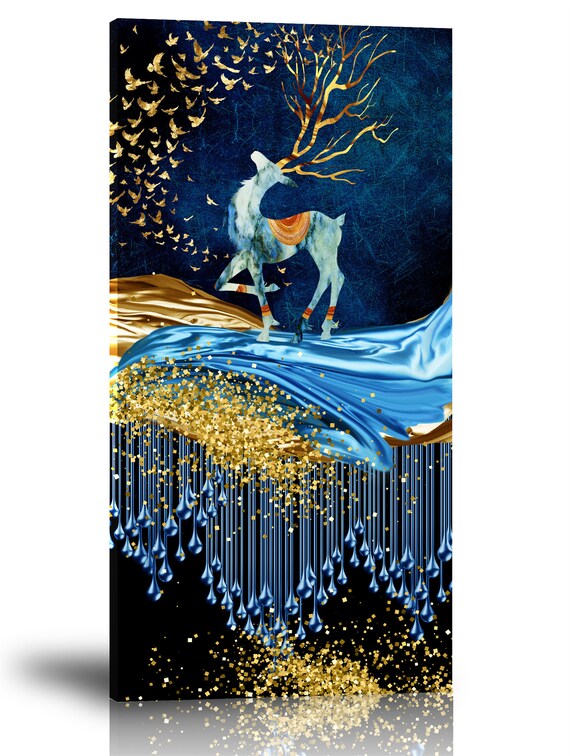The image is a tall rectangular canvas depicting a uniquely artistic scene. At its center is a light blue reindeer adorned with gold accents on its feet and back. The reindeer has grayish cream antlers that transition seamlessly into golden birds, which appear to be flying off into the top left corner. A dramatic interplay of metallic blue and gold waves flows through the middle of the artwork, with the blue wave originating from the right and the gold wave from the left side. Beneath these waves, golden specks and crystal blue teardrop-like droplets cascade down, creating an impression of intertwining elements. The background is a rich royal blue at the top, resembling a night sky, and transitions to black towards the bottom, scattered with more gold sparkles that further embellish the scene. This detailed composition blends elements of fantasy and nature in a strikingly creative manner.